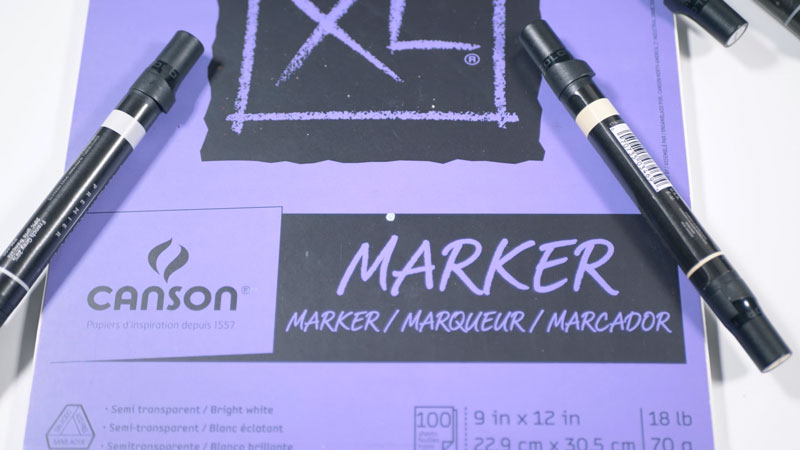This detailed image features a lavender-colored notebook prominently displaying the word "Marker" at the top in light purple, along with its translations "Markador" and "Marquer." Near the top, encased within a black square that mimics the texture of chalk, is the size indicator "XL." Towards the middle of the notebook, there's the company logo "Canson," which consists of the brand name below two stylized swirly lines. The lower portion of the notebook specifies its dimensions as 9 inches by 12 inches (22.9 cm by 30.5 cm) and its weight as 18 pounds (70 grams). Resting atop the notebook are three black markers, all neatly arranged. The entire composition is presented at an upright angle.